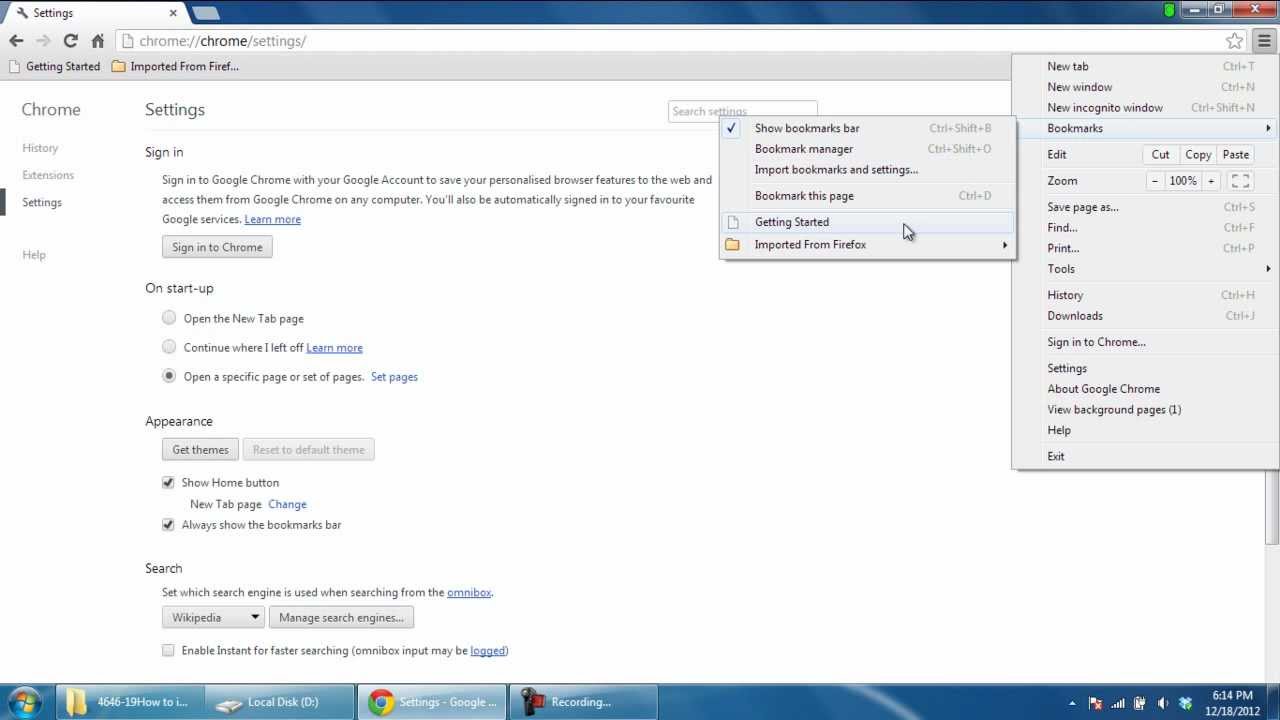Here’s a detailed and cleaned-up caption for the image:

---

The screenshot captures the Chrome settings page with a white background. The URL in the browser's address bar is bolded and reads "chrome://settings/". The "Getting Started" section appears to provide options to import data from possibly Firefox, abbreviated as "F-I-R-E-F...". Below, the "Chrome History" and "Extension Settings" are denoted with black lines. A "Help" section is present alongside a search box.

The page prompts the user to sign in for more personalized settings with a link labeled "Learn more" in blue text at the end. There's a gray rectangle with the option to sign in to Chrome.

Under the "On Startup" section, there are three radio button options:
1. "Open the New Tab page"
2. "Continue where you left off"
3. "Open a specific page or set of pages", with a "Set pages" link in blue text.

The radio button for "Open a specific page or set of pages" is selected.

In the "Appearance" section, there are options to "Get themes" and "Reset to default theme," with the latter option appearing grayed out and faint.